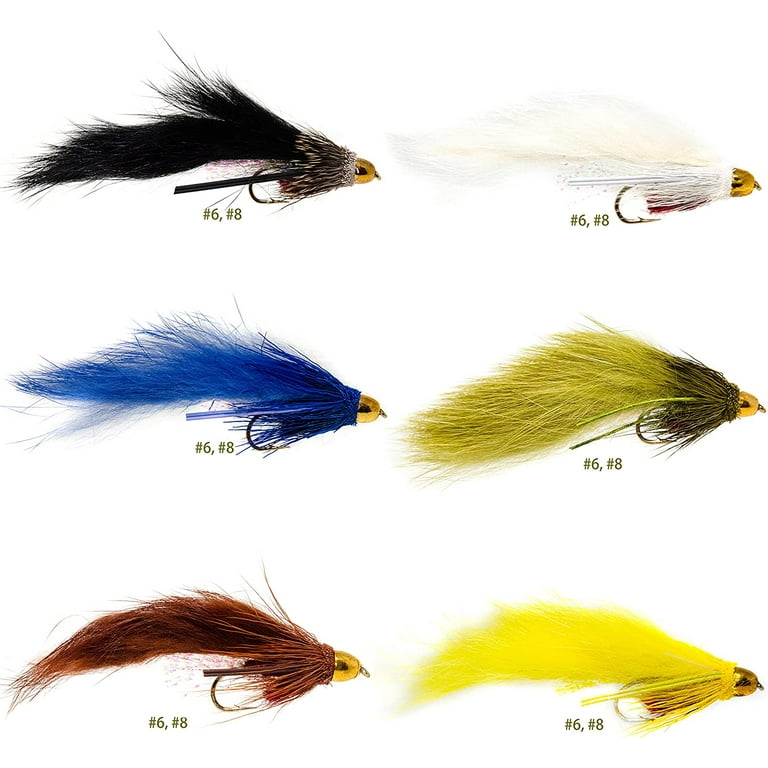This image showcases six different fishing lures arranged against a white background, each with numbered labels "6" and "8" beneath them. All lures share a similar design, featuring fuzzy materials resembling animal tails or feathers and are oriented with their ends facing to the left and a gold cap towards the right, from which a hook dangles. The top left lure is black with a gray neck and a yellow head. The top right lure is white with a slightly red-tinted neck and a yellow head with a black eye. The center left lure is blue with a darker blue neck and a yellow head. The center right lure is a mustardy darker yellow with an olive green neck and a yellow head with a black eye. The bottom left lure is brown, featuring a slightly lighter neck and a yellow head. Lastly, the bottom right lure is a vivid bright yellow with a hint of red in the neck and a darker yellow head.